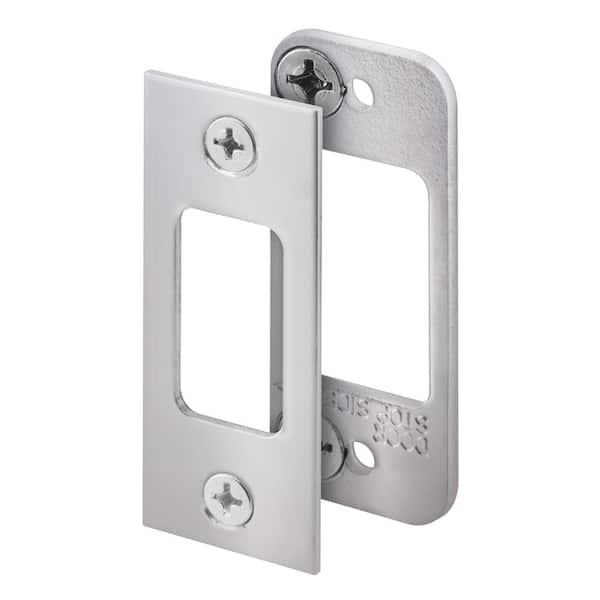The photograph depicts a pair of interlocking faceplates, designed for a door latch or similar application. The foremost plate is white and rectangular with a central, rectangular cutout featuring rounded corners. It has two prominent screws, one at the top and one at the bottom, designed for attachment. The accompanying plate, also white, features stamp markings at the bottom and two screws on the left side, with holes to align with the screws from the first plate, indicating they work in tandem. Both components are presented on a white background, highlighting their metallic, silver-gray finish. The image is an angled, close-up shot, clearly detailing the screws and the precision fit of the components.